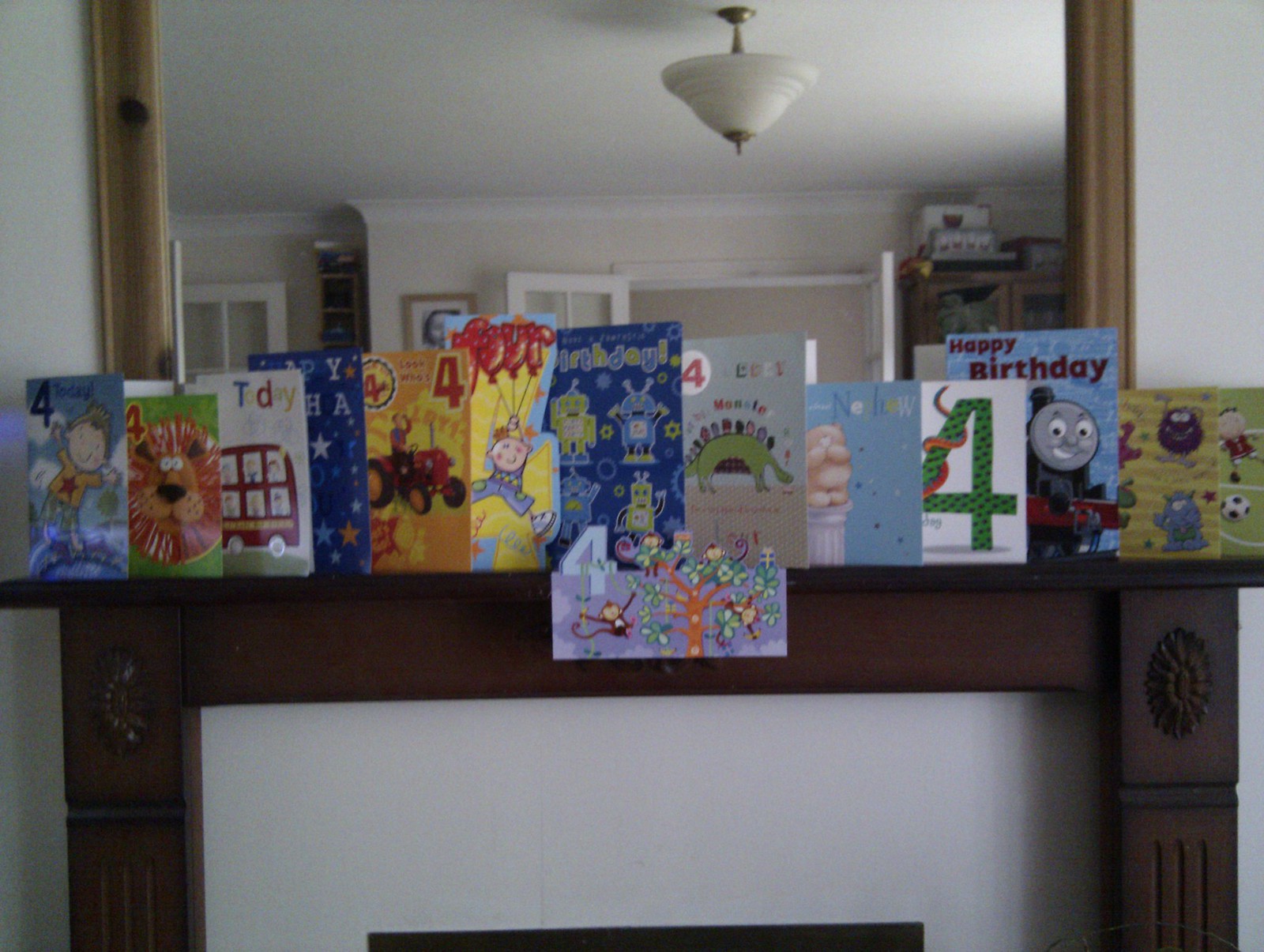This photograph captures a dark wooden mantelpiece adorned with a vibrant collection of twelve children's birthday cards, predominantly featuring the number four and playful themes. Among the cards, notable designs include Thomas the Tank Engine, a red tractor, a red taxi labeled "Today," a cartoon boy in a yellow t-shirt and green shorts with a star, a brown lion, aliens, a green dinosaur, and a blue card with red writing. Each card adds a unique touch of color and whimsy, suggesting a celebration for a four-year-old child. Above the mantelpiece is a large mirror reflecting the room. In the mirror's reflection, we see a white cone-shaped ceiling light with a gold hanging feature, white-framed French doors with glass panels, and a glass cabinet beside a CD shelf and a framed pencil illustration on the opposite wall. The room has a white ceiling and walls, contributing to a bright and airy ambiance.